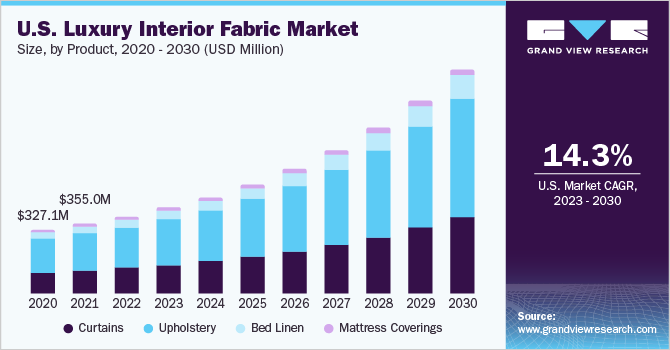The image depicts a detailed bar chart titled "US Luxury Interior Fabric Market" with the subtitle "Size by Product (2020-2030) in USD million." The chart, set against a light gray background and featuring a bluish line across the top, represents data from 2020 to 2030. Each bar in the chart is color-coded to indicate different categories: dark navy for curtains, darker teal for upholstery, light blue for bed linen, and pink for mattress coverings. The initial data points include 327.1 million USD for 2020 and 355.0 million USD for 2021, with each successive year showing an upward trend, culminating in the highest bar for 2030.

In the top right corner, there's the Grandview Research logo, a stylized "GVR" comprising a square with lines indicating the "G" and "R" and a triangle for the "V." Below the logo is the notation "14.3% U.S. Market CAGR (2023-2030)." The chart's source is listed as www.grandviewresearch.com.